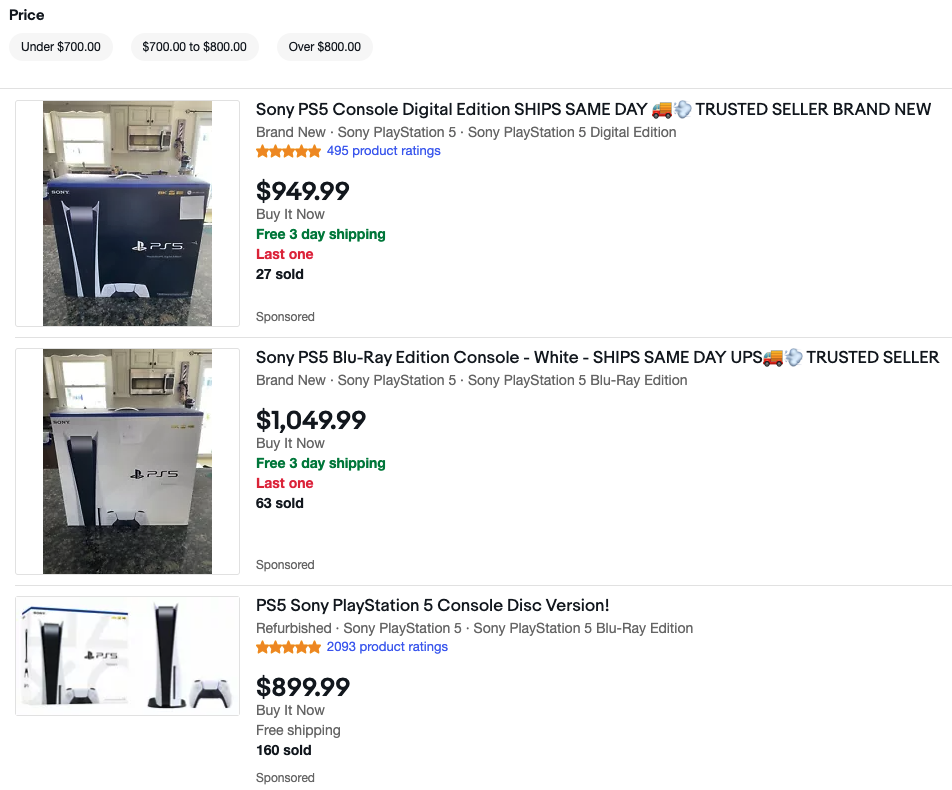This image is a detailed screenshot of a product comparison for various Sony PlayStation 5 (PS5) consoles from a trusted seller. 

In the first boxed listing, the featured item is a Sony PS5 Console Digital Edition, boasting a "ship same day" promise. It is described as brand new with a "Buy It Now" price of $949.99. The listing offers free three-day shipping, notes it is the last available item with 27 units already sold, and is marked as a sponsored advert.

The second boxed listing showcases a Sony PS5 Blu-ray Edition Console in white. This item also ships the same day from a trusted seller and is priced at $1,049.99 as the "Buy It Now" option. This listing includes free three-day shipping, highlights it as the last available item, and mentions that 63 units have been sold. It is also categorized as a sponsored post.

The third boxed listing provides a PS5 Sony PlayStation 5 Console Disc Version, explicitly marked as refurbished. This refurbished version of the Sony PlayStation 5 is available at a "Buy It Now" price of $899.99, includes free shipping, and has seen 160 sales. Like the other two, this is also a sponsored listing.

At the very top of the comparison, there is a price filter section containing three distinct categories: "Under $700," "$700 to $800," and "Over $800." In this screenshot, none of these price range options appear to be selected. All three listings are for different versions of the Sony PS5, emphasizing varied prices and conditions but uniformly indicated as sponsored.